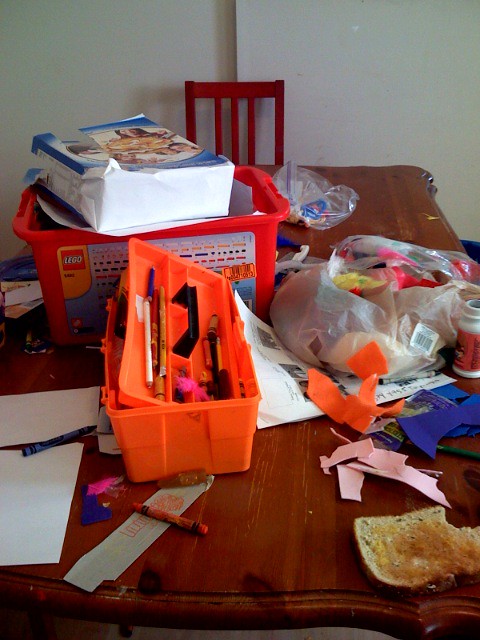The image depicts a cluttered, brown table covered with a variety of items. On the table, there is a partially toasted piece of bread with a bite taken out of it. Scattered around are blue and orange crayons, colored pencils, pieces of paper in various colors—primarily purple and blue—and several crayon boxes. Notably, one box is orange and likely serves as the crayon container. A larger box with a Lego logo sits on the table; however, it appears empty, save for a torn, white piece of paper atop it. Toward the right side of the table, there is a bag filled with indistinct items, adding to the general messiness. Behind the table, a white wall serves as the backdrop. A chair is positioned on the opposite side of the table. The scene is one of creative chaos, with various art supplies and remnants scattered about.